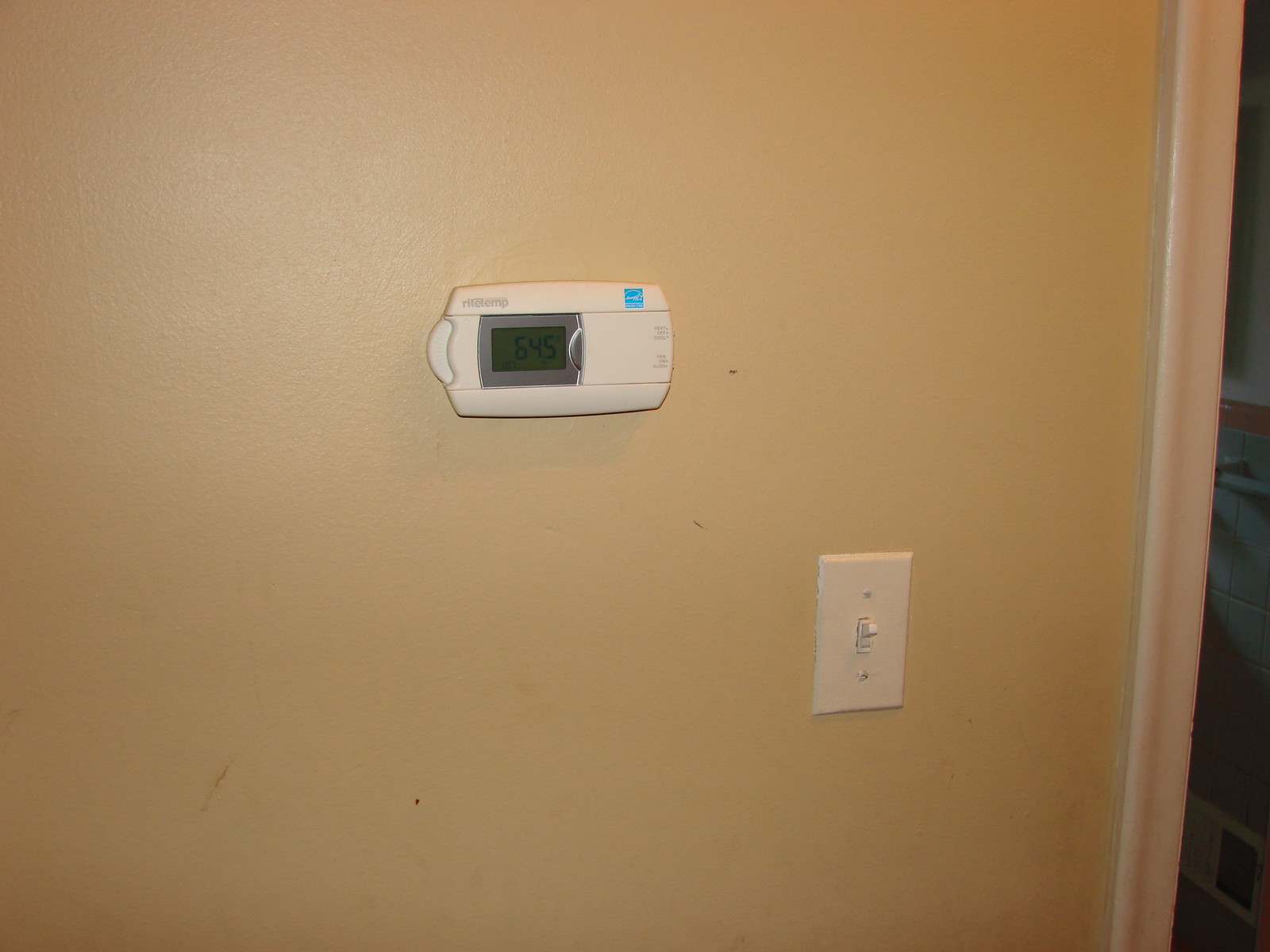In this photograph, a white light switch and an air conditioning control unit are mounted on a light orange or light tan wall with a smooth, painted surface. The light switch, positioned towards the right side of the image, has a knob in the middle of a slightly protruding white rectangular plate, and is currently toggled to the "on" position. To the left of the light switch, at the middle of the frame, is the air conditioning control unit. The unit is a white triangle with its long side oriented horizontally and the short side vertically. In the middle of this unit, slightly to the left, there is a small gray box displaying the numbers "645" in illuminated black text. At the top right corner of the control unit, there is a black square with white text inside. Extending from the center of the left side of this unit is a curved button. 

On the right edge of the image, a white door frame is visible, leading into what appears to be a dark bathroom with gray tiled walls. An illumination from a nearby light source casts a white glow on the wall near the air conditioning unit.